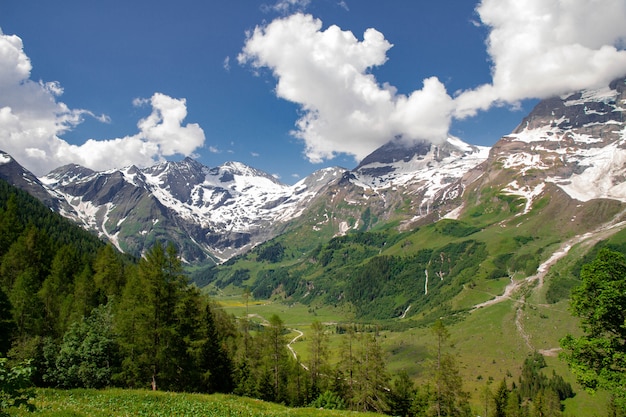The real-life photograph captures a breathtaking alpine landscape on what appears to be a bright, sunny summer day. The image is landscape-sized, beginning with a lush valley in the foreground filled with vibrant green grass, bushes, and towering evergreen trees. Towards the middle, the terrain begins to ascend into hills, leading up to a towering mountain range.

The mountains dominate the background, their peaks capped with remnants of snow that contrast starkly against the vivid blue sky. The sky itself is dotted with fluffy white clouds, some of which descend to obscure parts of the highest peaks, suggesting a high elevation, possibly between 10,000 to 12,000 feet. 

A path can be observed winding through the greenery, leading the eye toward the more desolate, rocky upper slopes of the mountains where the trees thin out and eventually disappear. The mountain peaks are rugged and grey, standing as a formidable backdrop to the lush, healthy valley below. In the distance, there are hints of a house or structure, adding a touch of human element to the otherwise natural scene.

The landscape appears serene and pristine, possibly located in a region like Switzerland or Austria, exhibiting the transitional beauty from a fertile valley to the stark, snow-kissed mountaintops.